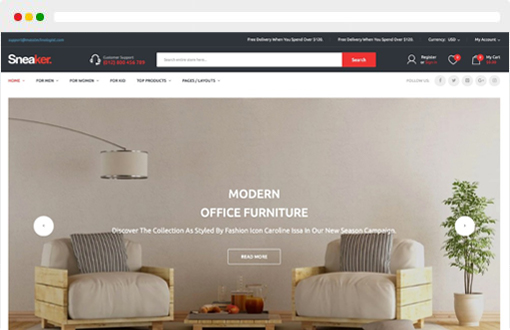The image features a user interface with various visual elements and a room interior. At the top, a light gray box contains three colored circles on the left side: a red circle, a yellow circle, and a green circle arranged vertically. Below this sits a white text box, which is empty, followed by a slightly blurry black border at the top containing text that is difficult to decipher due to the blur. Visible on the left side of this black box is the word "Sneaker," with "Snea" in white letters and "ker" in red letters.

Further below, there is a white search bar accompanied by a red button. To the right of the search bar, a notification bell icon displays a red notification dot, followed by a heart icon also with a red notification dot. Underneath these elements lies a menu, which appears to contain links to social media.

The lower part of the image is dominated by a large photograph of a room characterized by a gray wall and a ceiling lamp descending from the left side. The room features two chairs with notably thick seat cushions and armrests constructed from three stacked 2x4s, emphasizing a robust and rustic design.